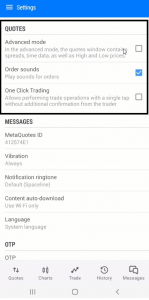A screenshot of a stock market trading app's settings page is displayed. Despite being slightly blurry, several key features can be discerned. The user has accessed the "Advanced Mode" which is highlighted, indicating a preference for more complex trading tools. The "Order Sounds" option is also selected, allowing the user to receive audio notifications, such as jingles or bells, when orders are executed. Below these settings, there are tabs labeled "Trade," "History," "Messages," and "Charts," suggesting comprehensive functionality for tracking and managing trades. The interface is primarily white and gray, creating a clean, uncluttered background, with a blue header bar at the top demarcating the settings menu.